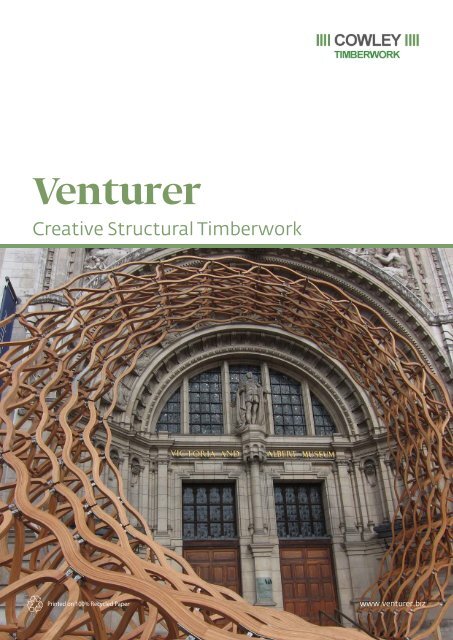The poster image features a detailed color photograph of the entryway to the Victoria and Albert Museum. The building's exterior is constructed from light gray stone with two brown wooden doors, each with windows above them. Above the doors, gold text reads "Victoria and Albert Museum," identifying the location. The entrance is framed by an arched structure, which includes a small statue on a pediment centrally positioned above the doors. Surrounding the entrance is an elaborate, circular, trellis-like sculpture made of interlocked, wavy wooden pieces that are light brown in color. These pieces form a swirling design that begins at the bottom right door and extends outward and around the entryway. At the top right corner of the image, the text "Kauley Timberwork" is printed, while the bottom left corner contains green text that reads "Venturer Creative Structural Timberwork".